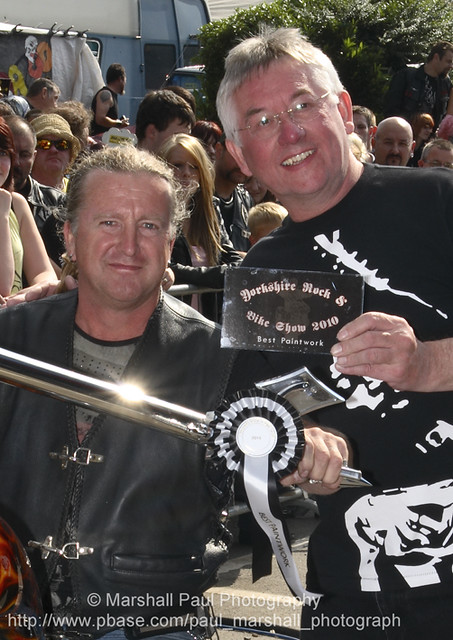In this vibrant outdoor event photograph, two men are prominently posed in the foreground. The man on the right, displaying a friendly smile, has greying hair and wears glasses. He's dressed in a black and white t-shirt and is holding a transparent plaque that reads "Yorkshire Rock and Bike Show 2010 Best Paintwork." In his other hand, he holds a silver bar adorned with a black and white ribbon. The man on the left, with brown hair tied back and clad in a leather jacket over a t-shirt, stands confidently beside him. A large crowd can be seen in the background, suggesting a lively event atmosphere. At the bottom of the image, the text reads "Marshall Paul Photography, http://www.pbase.com/.paul-marshall-photograph," indicating the photo’s attribution.